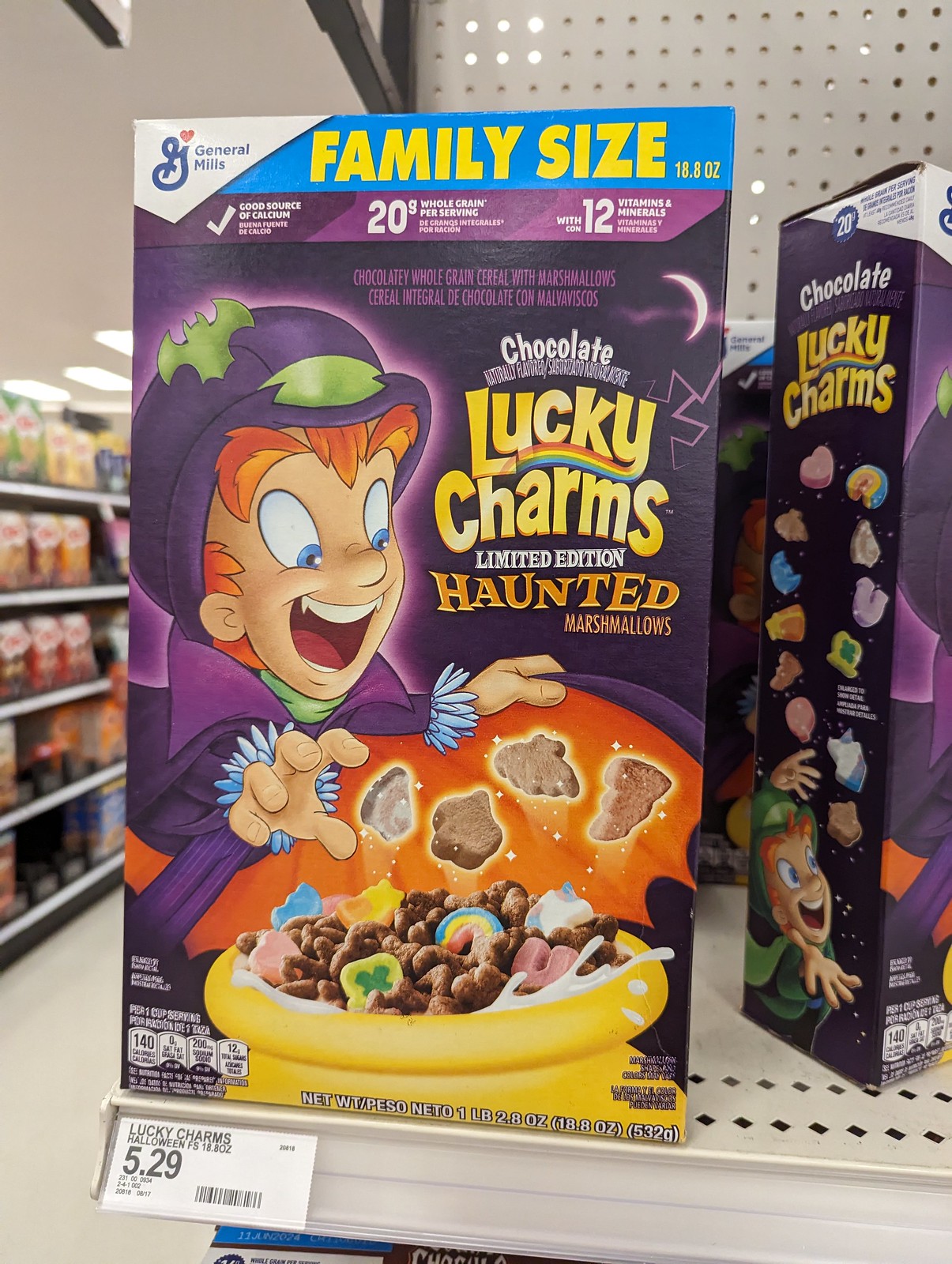The image depicts a white steel shelf in a grocery store, displaying several boxes of General Mills' Limited Edition Haunted Lucky Charms cereal. The boxes are family-sized, containing 20 grams of whole grains per serving, 12 essential vitamins and minerals, and each box boasts a good source of calcium. The front of the box is predominantly purple, with a distinctive Halloween theme featuring the iconic leprechaun character. He is depicted with red hair, wearing a black hat adorned with a green bat and additional spooky elements like a bat and possibly a witch's hat. His outfit includes a green shirt with pointy cuffs. The leprechaun is intently staring at a yellow bowl filled with chocolate Lucky Charms cereal mixed with colorful marshmallow shapes including ghosts. The General Mills logo occupies the top left corner, and the price tag on the shelf indicates that the cereal is being sold for $5.29. In the background, other grocery items are faintly visible, contributing to the typical grocery store ambiance.